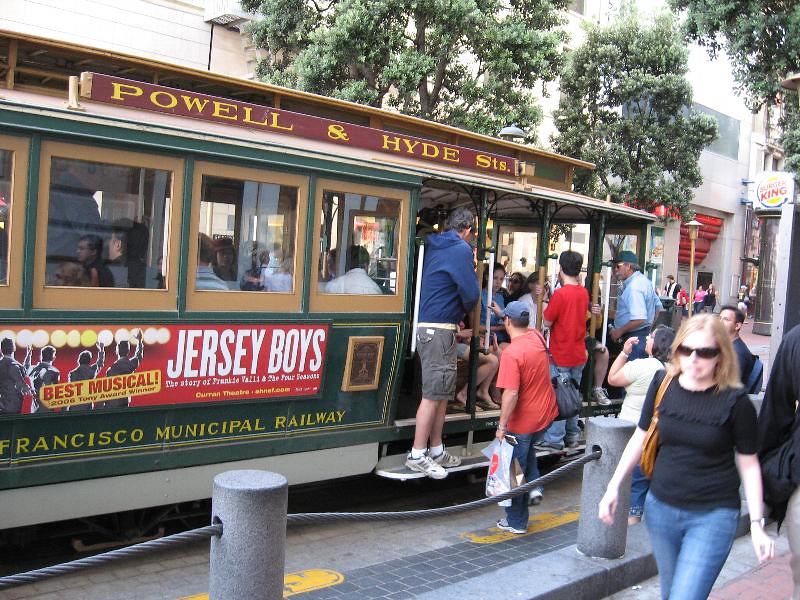The photograph is a vivid depiction of a lively San Francisco street on a pleasant day. Dominating the scene is a green and brown San Francisco trolley, marked with "Powell and Hyde Streets" in yellow letters on a burgundy background. The trolley is adorned with an advertisement for the musical "Jersey Boys," labeled "Best Musical," and further identified as part of the Francisco Municipal Railway. Passengers are visible inside the trolley, with several people in the process of boarding, gripping the poles and stepping onto the rail. The background features a mix of urban and natural elements, including a partially visible building with several windows, and trees with green foliage. Prominent in the center-right of the image is a sign for Burger King. The street and sidewalk are bustling with people, including a blonde-haired woman in jeans and a black t-shirt, distinctively wearing large black sunglasses, walking towards the camera, detached from the trolley activity. Cement poles connected by ropes line the sidewalk, adding to the structured city atmosphere.